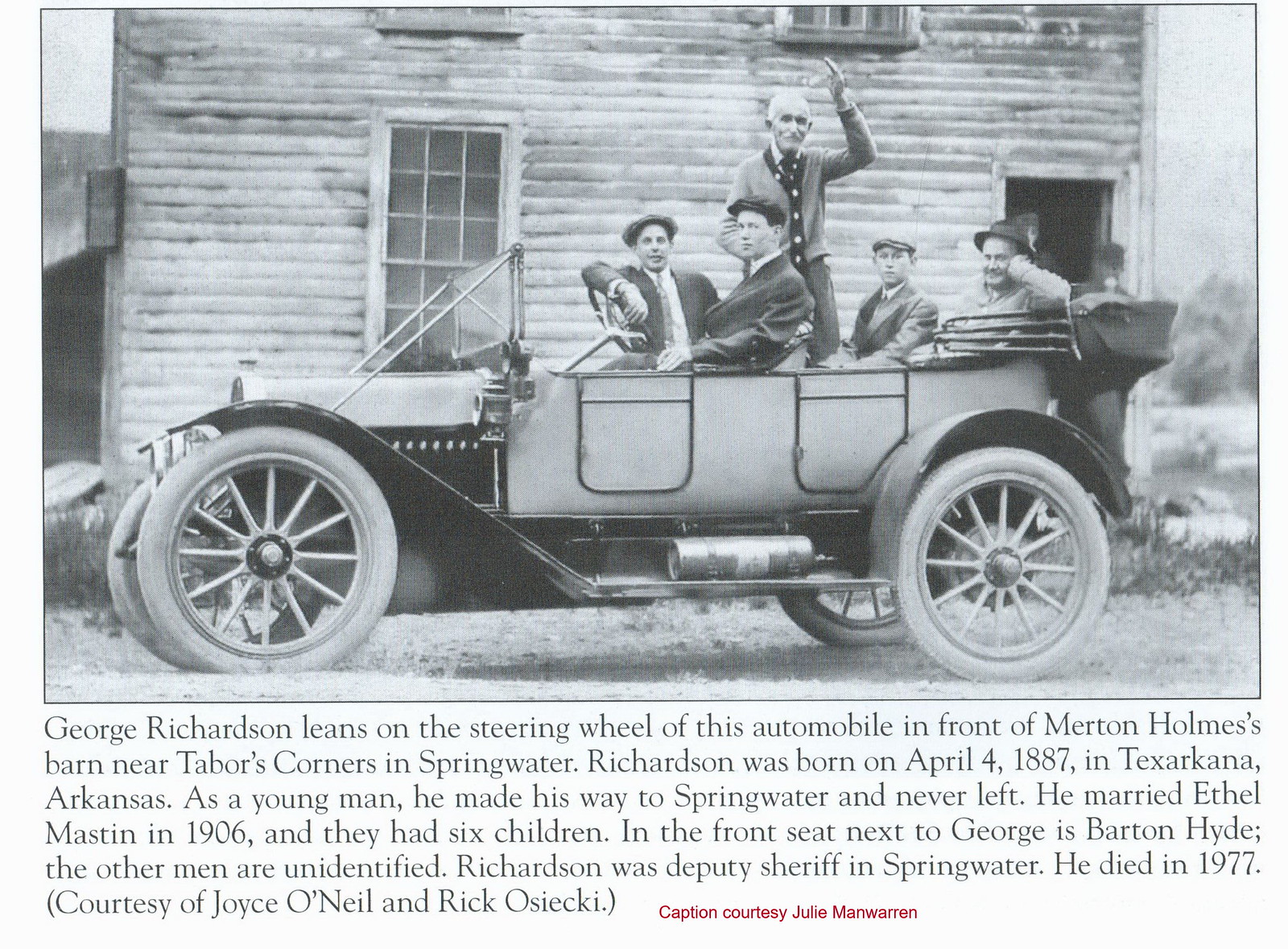The black-and-white photograph captures a scene from an era long past, showcasing an old-school convertible car with five men. In the front seat, George Richardson leans on the steering wheel, with Barton Hyde next to him. Both men, likely in their mid-30s or 40s, are dressed in hats and suits with ties. Seated in the back are two more men: one appears to be a young adult or teenager, and the other, alongside them, is also in formal attire. Another elderly man, characterized by his white hair and raised left arm, stands up in the car. They are positioned in front of Merton Holmes's barn near Tabor's Corner in Springwater. Born on April 4, 1887, in Texarkana, Arkansas, George Richardson moved to Springwater as a young man, married Ethel Mason in 1906, and served as the town's deputy sheriff until his death in 1977. The caption, provided by Joyce O'Neill and Rick Osiecki, ends with the note that Richardson's story was courtesy of Julie Manwaran.